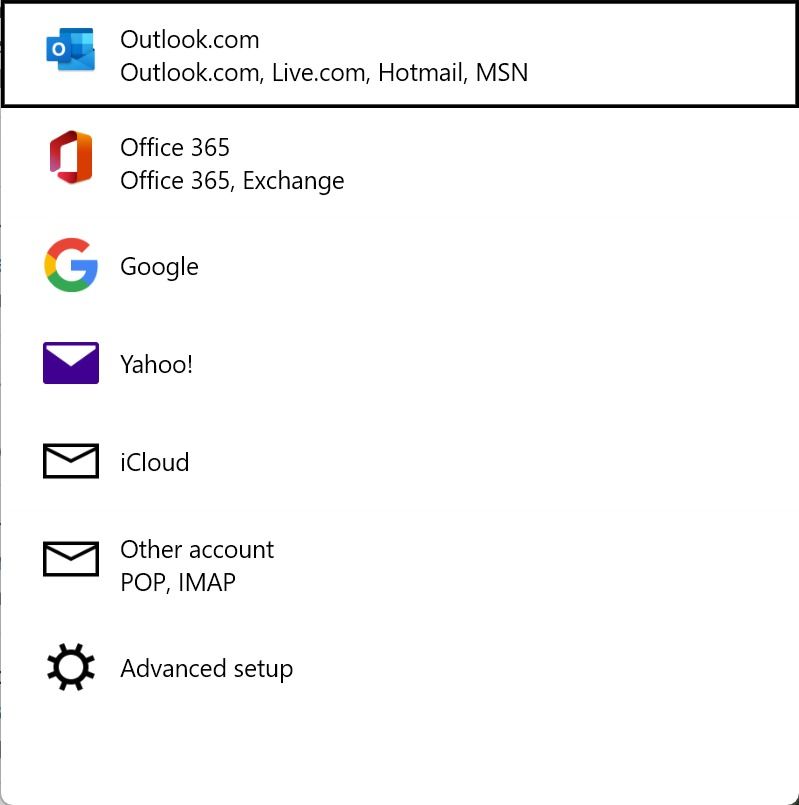The image displays a detailed list of various email sources arranged in a vertical, top-down format. Each source is accompanied by its corresponding icon situated to the right. The list is prominently bordered by a black outline, separating it from the surrounding content. At the very top of the list is "Outlook.com," followed by another entry for "Outlook.com," then "Live.com," "Hotmail," and "MSN." Below these, additional categories are listed starting with "Office 365," followed by "Exchange," "Google," "Yahoo!" with an exclamation mark, "iCloud," "Other Accounts," and finally "POP, IMAP," representing the various types of other accounts. At the end of the list lies "Events Setup." Each of these email sources is represented by distinct icons to visually distinguish them. The overall layout is clear and organized, making it easy to identify each email source and its related icon at a glance.